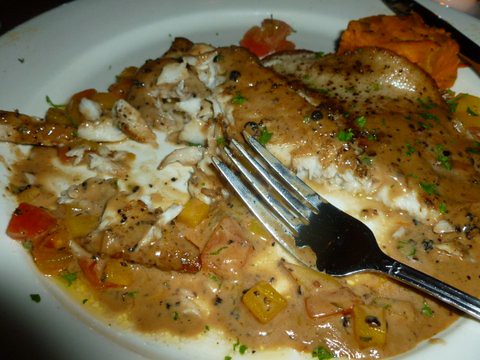This image depicts a plate of partially-eaten food, with a focus on various elements making up the messy scene. The white plate is close up, showcasing a mix of brown and white food that appears to be grilled fish or meat, covered in a light brown gravy. Among the mixture, there are small, cut-up vegetables including yellow chunks that might be peppers, orange and red pieces, and specks of black pepper or grill marks. There are hints of chives or some other green garnish scattered on top. A fork lies across the lower right part of the plate, smeared with food, and in the upper right corner, there is another utensil partially visible next to an orange mass that could be a piece of sweet potato. The plate's rim is notably dirty, with food specks spilling over its edges, enhancing the overall untidy appearance of the meal.